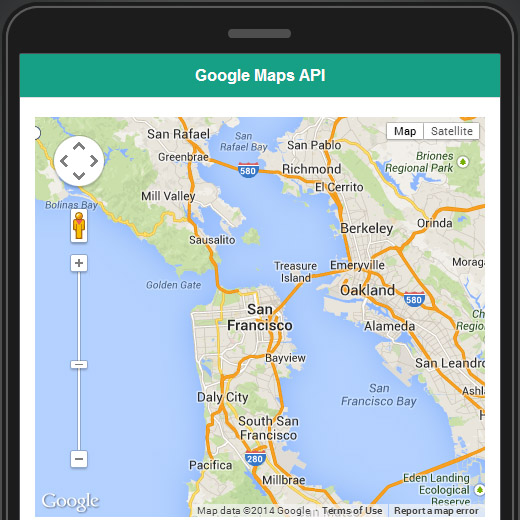This image depicts a Google Map displayed on a phone screen. The interface lacks typical phone icons at the top, suggesting a focus on the map itself. A green border at the top indicates the use of the Google Maps API. The map features a detailed view of the California area, prominently showing San Francisco, the Bay Area, Sausalito, and the Golden Gate Bridge. Major roads are highlighted in a gold color, including interstate highways 580 and 280, and various cities such as Daly City, Pacifica, and Millbrae are clearly labeled.

A zoom slider on the interface allows for interactive scaling of the map, enabling users to zoom in and out. In the lower-left corner, the familiar Google logo appears in white text. The map also shows Boneless Bay with additional icons and features. One such icon is an image of a person in a solid tan color, positioned below a white circle containing a diamond-shaped box with breaks on each side. The top right corner offers options to switch between "Map" and "Satellite" views, enhancing the map's functionality for diverse user needs.